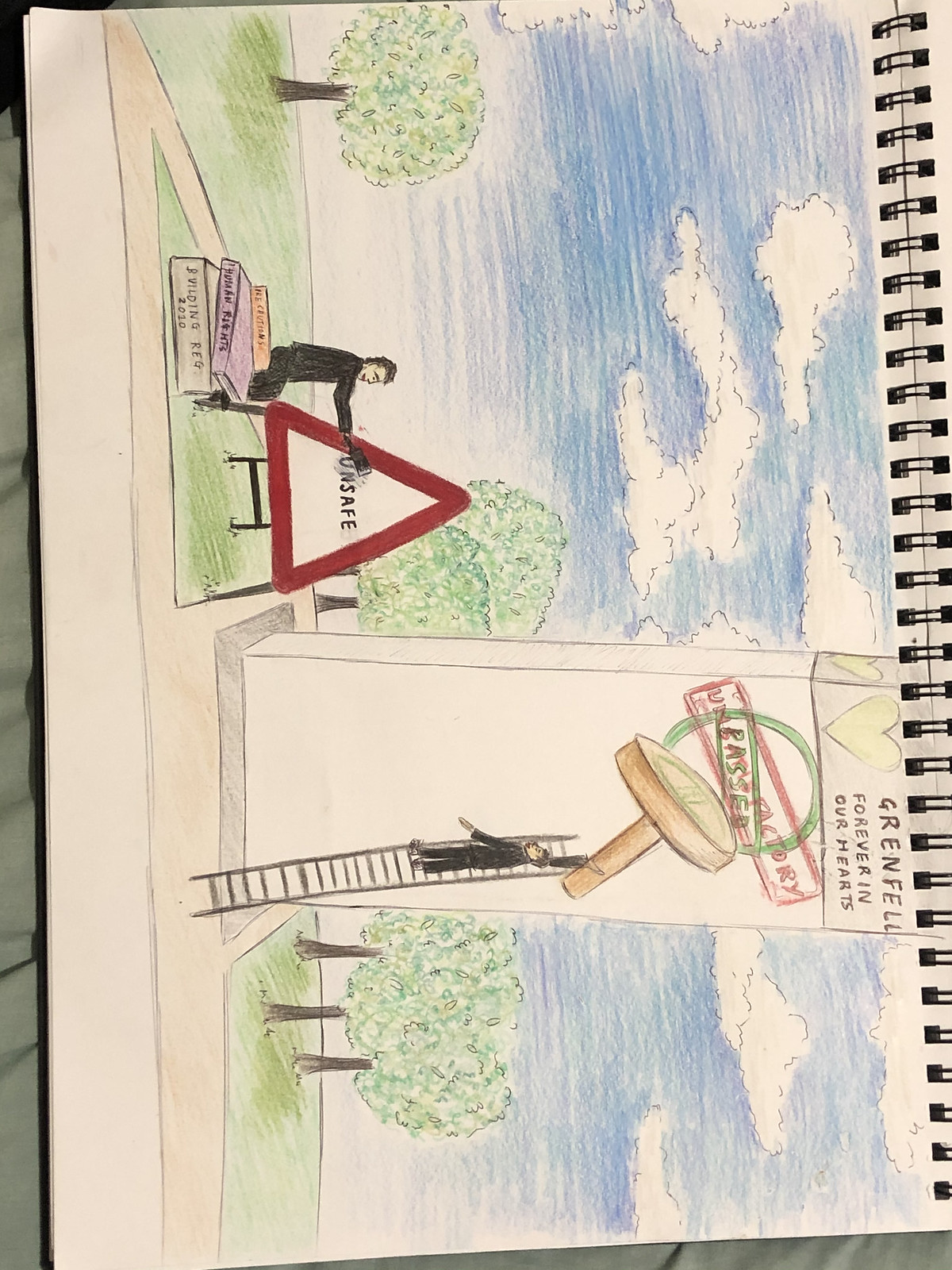This detailed sketch on plain white paper in an artist's sketchbook captures a park scene with vibrant colors using colored pencils and outlined in plain pencil. The sketch is oriented horizontally, reminiscent of a landscape view. Dominating the right side of the image is a serene blue sky interspersed with white clouds, while the left side features a sprawling green lawn in a light yellow hue. Five perfectly round trees with lush green leaves punctuate the background.

In the foreground, a person dressed in black sits on a block beside a triangular caution sign marked with the word "UNSAFE." This individual appears to be interacting with the sign, possibly altering the inscription. A stack of school books rests nearby. Further to the right, a large rectangular white monument stands tall, with another figure dressed in black perched on a ladder, seemingly making modifications to the monument with a green colored pencil. Above this scene, the poignant inscription "Greenfield forever in our hearts" is flanked by a yellow heart, suggesting a tribute to a cherished place, possibly a school or community landmark.